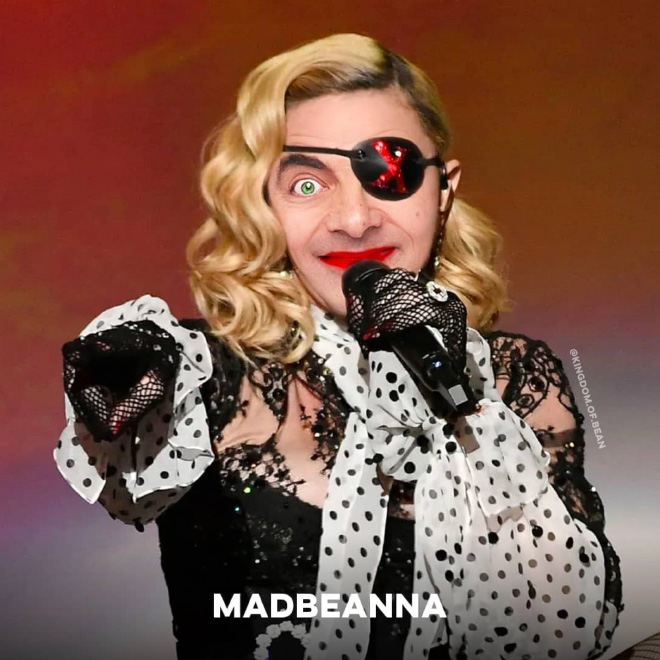In the image, the character resembling Mr. Bean is dressed in drag as Madonna. He has long, curly, blonde hair cascading down to his shoulders. His face features a bright green artificial eye while his left eye is concealed by a black eye patch marked with a red 'X', reminiscent of a pirate. His expression is accentuated by vivid red lipstick. He is adorned in iconic 80s Madonna-style attire, including lacy mesh gloves and a black outfit with white, sheer, poofy sleeves dotted with black polka dots. The text at the bottom of the image reads "Mad Beana" in centered white font. The backdrop is a dull reddish-orange hue. Additionally, there is a small copyright notice to his right that says "@kingdom.of.bean."